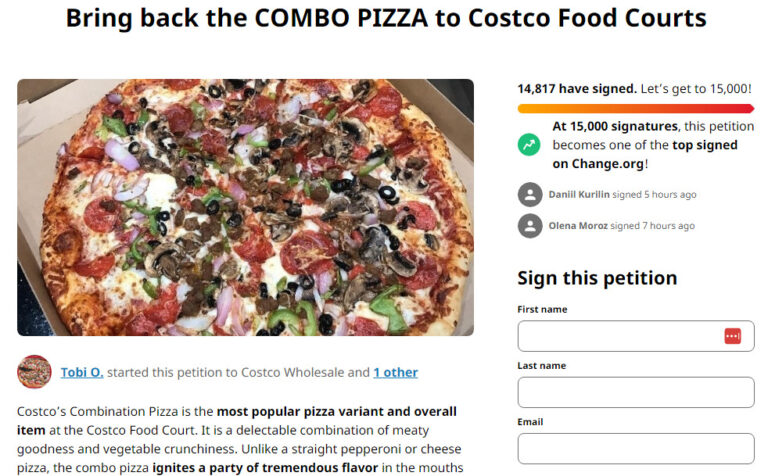**Caption:**

A vibrant petition urging Costco to bring back their beloved combo pizza takes center stage. At the top, bold text reads, "Bring Back the Combo Pizza to Costco Food Courts." To the left, a mouthwatering image of a large combo pizza fills a cardboard box. The pizza is loaded with a variety of toppings, including pepperonis, olives, ham, onions, peppers, a rich tomato sauce, and a perfectly baked crust.

On the right side, a progress tracker with a reddish-orange bar reveals that 14,817 supporters have already signed, edging closer to the goal of 15,000 signatures. An annotation below highlights, "At 15,000 signatures, this petition becomes one of the top signed on Change.org."

Further details are provided with a green circle and white up-arrow icon, indicating a trend of upward momentum. Beneath this, small icons featuring recent signatories such as Daniel Turin and Alina Moraes are displayed, indicating their support five and seven hours ago, respectively. 

Below the pizza image, there's a circular icon with a picture of the pizza, accompanied by the text: "Toby Oh started this petition to Costco Wholesalers and one other." Supporting text emphasizes the importance of the combo pizza, describing it as Costco's most popular food court item. The combination pizza, celebrated for its blend of meat and vegetables, offers a unique flavor experience unlike conventional pepperoni or cheese pizzas. 

To the left, a sign-up section is available for new supporters, requesting their first name, last name, and email to join the cause.